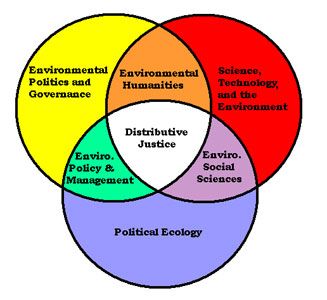This image features a detailed Venn diagram composed of three intersecting circles with distinct colors and shared sections, all containing informative black text. The top left circle is highlighted in yellow and prominently labeled "Environmental Politics and Governance." It shares a brown and white section on the right side with the top right circle. This top right circle is mainly red and labeled "Science, Technology, and the Environment." Both top circles share a purple section at their base with the bottom circle. The bottom circle is primarily blue and is labeled "Political Ecology," with portions connected to the other two circles. Specifically, the shared sections are: brown for "Environmental Humanities," white in the center for "Distributive Justice," green on the left side connecting the lower and left circles for "Environmental Policy and Management," and purple for "Environmental Social Sciences." This Venn diagram visually represents the intersections between different disciplinary focuses within environmental studies.